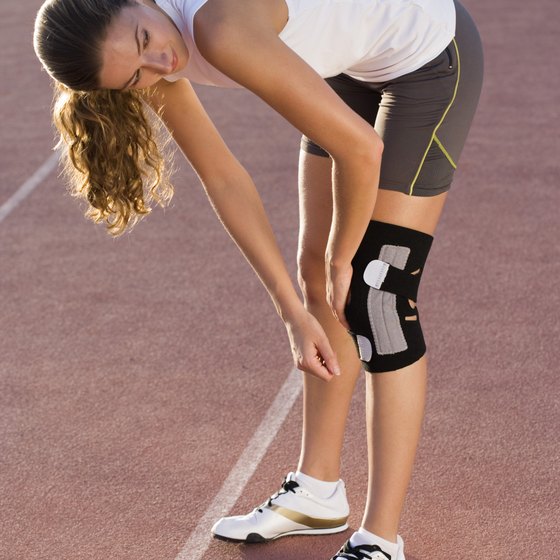In the vivid photograph, a female athlete, clearly a track runner, occupies the center of the frame, which is a vertical rectangle almost resembling a square. The action takes place outdoors on a running track, evident from the distinctive red-tinted textured ground adorned with two parallel white lines marking the lanes. The woman, who has brown hair, is dressed in short grey bike shorts with hints of yellow and a sleeveless white tank top. She is adorned with white sneakers featuring black and gold accents, including a notable gold line. The focal point of her posture is her bending stance, where she is leaning forward, attending to a gray and black knee brace with white latches on her left knee, touching and adjusting it. The combination of black, gray, white, gold, brown, tan, yellow, and a pinkish-brown skin tone colors paints a detailed and dynamic image of a dedicated athlete in the midst of her pre-run routine.